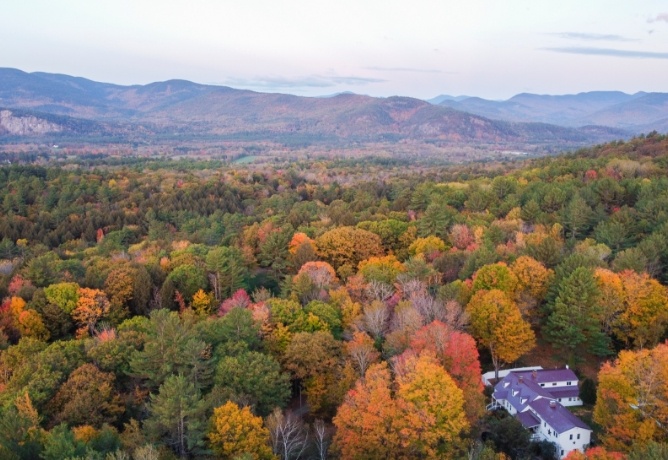This aerial autumn photograph captures a breathtaking landscape dominated by a vibrant sea of trees in various shades of green, gold, red, and muted orange. The dense forest stretches unbroken from the immediate foreground all the way to a distant mountain range that gently slopes from left to right. The sky is a grayish hue, dotted with a few clouds, adding to the serene atmosphere. Nestled in the bottom right corner of the image is a small, isolated building with white siding and a maroon-brown or dark purplish roof, appearing to be two to three stories tall. It features numerous rectangular windows and has a paved pathway or driveway leading away from it. The structure appears to be a house or possibly two closely positioned buildings, giving an L-shaped impression from the aerial view. There are no other visible structures or roads, emphasizing the building's solitude amidst the enveloping autumn foliage, with a few trees in the foreground already starting to shed their leaves.